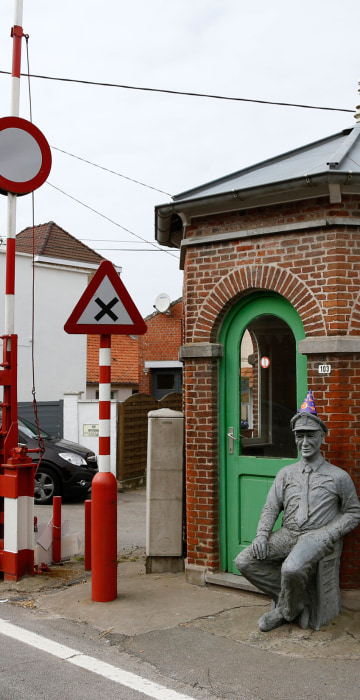In this photograph, taken during an overcast day with a gray sky background, a detailed scene at what appears to be a historical crossing or toll gate is depicted. Dominating the scene is a red-bricked building featuring a Palladian arch and a prominent green door. To the right of the green door sits a statue of a man, possibly representing a World War II service member, distinguished by his hat, shirt, and tie. The statue is bronzed and depicts the man sitting with one hand in his pocket and the other on his thigh. 

In front of the building, to the left of the doorway, stands a tall red-and-white striped post with a red triangular sign marked by an X in the center, indicating a railroad crossing. Multiple power lines crisscross the sky overhead. Additionally, a black car is parked near the building, contributing to the contemporary feel of the scene despite the historical elements. The combination of these features – the brick structure, the prominent green door, the commemorative statue, and the distinctive crossing signage – suggests that this location may serve as a museum or a historical landmark commemorating important past events or figures, possibly in a British or European context.